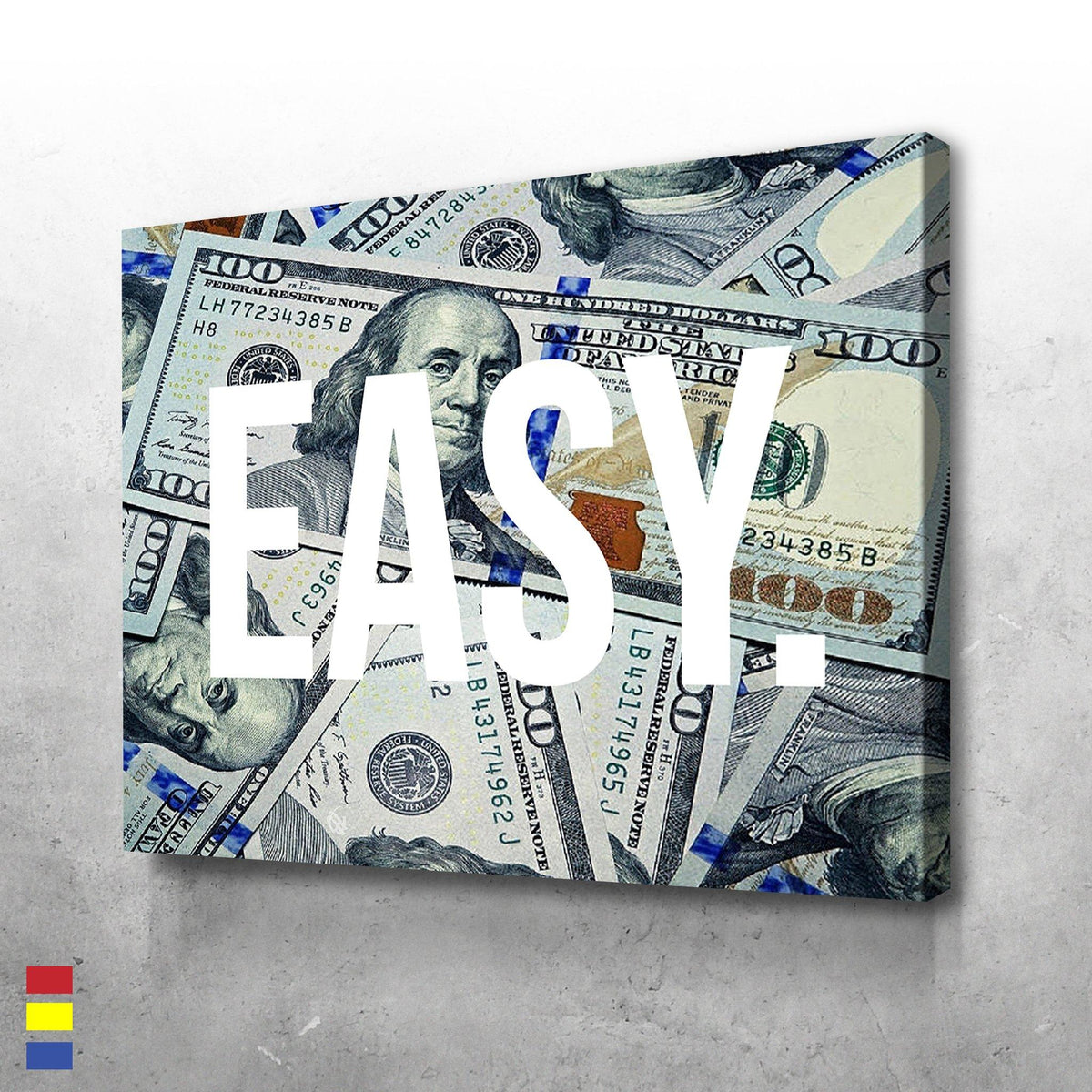In the image, a canvas is prominently displayed against a gradient gray wall. This canvas showcases a design featuring multiple $100 bills, meticulously arranged and vividly colored to resemble actual currency. Each bill is detailed with greenish-gray hues, the face of Benjamin Franklin, gold "100" markers in the corners, and distinctive blue security strips. Centered across the canvas, the word "EASY." is boldly written in large, all-capital white letters. Additionally, the canvas is likely wrapped around a brown wooden frame. The gradient wall darkens from white at the top to darker gray at the bottom, where it features black and white smudges. In the bottom left corner, there are three small rectangles aligned vertically in red, yellow, and blue.